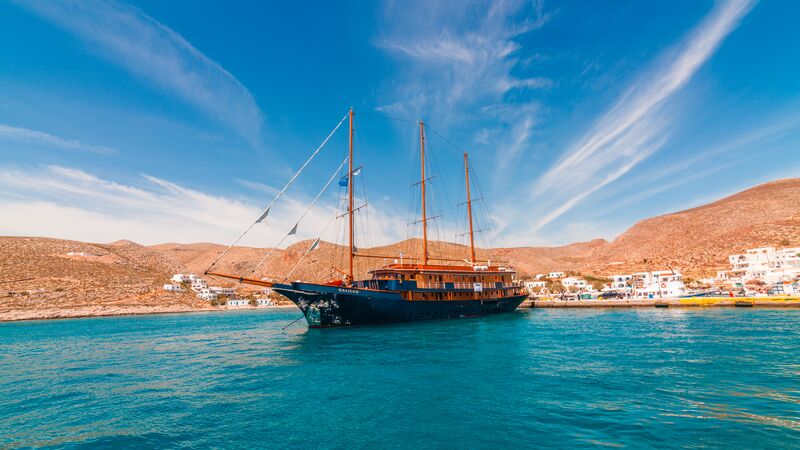The image depicts a large sailboat navigating a blue ocean under a mostly clear sky with light clouds. The sailboat, a striking mix of dark blue and brown, features three tall brown masts and has a prominent plank at its bow. The backdrop showcases towering, barren brown mountains that encircle a city, adding to the scenic beauty of the photograph. Despite the detailed urban and natural elements, no text is visible within the image. Hints of white and green add subtle color variations to the predominantly blue and brown scene.